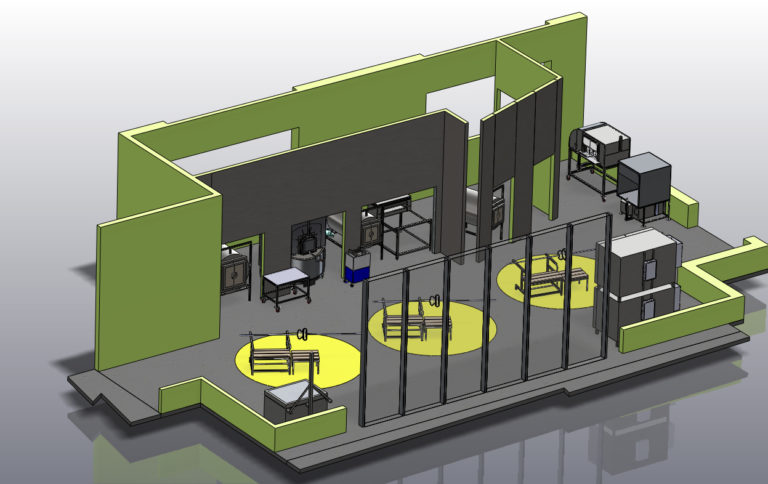This is a detailed 3D computer rendering of an office space. The floor is black, providing a stark contrast to the single visible green wall adorned with black accents. In the middle of the room, there are three large yellow circles on the floor, each featuring a bench placed precisely on top of them. To the right side of the diagram, there's an area designated for floor-to-ceiling windows framed with black accents, giving an impression of openness and light. Toward the back left of the room, five doorways can be seen, each leading to separate office spaces. The back wall appears gray with small cut-out areas near the bottom, possibly designed to accommodate cables or other utilities. Additional gray square or rectangular objects are scattered throughout the space, though their specific functions are unclear. The background of the rendering is kept basic and blank to focus attention on the layout and design details of the room. The overall design combines open space with individually marked areas, potentially indicating a versatile and functional office environment.